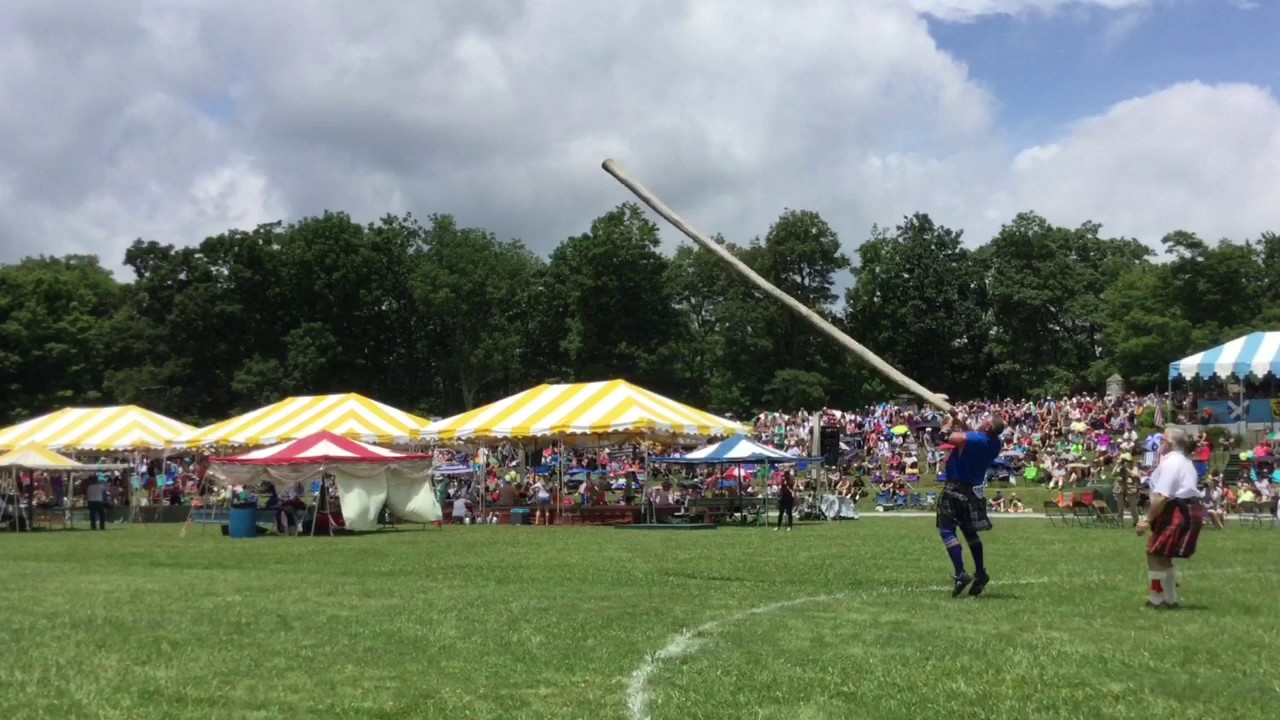The image depicts a lively outdoor event, possibly a traditional Scottish Highland Games held in a village or rural area. Central to the scene are two men in kilts, one in blue and the other in a red kilt and white t-shirt. The man in blue appears to be holding or about to throw a large wooden pole, suggesting he is participating in the caber toss, a classic Highland sport. Positioned a few feet behind him, the man in the red kilt seems poised to assist or ensure safety during the throw.

Surrounding them, a diverse crowd of spectators is visible, some seated on a grassy bank under the sun, while others find shade beneath numerous canopies. These canopies are vividly colored—with several yellow and white striped tents being the most prominent, accompanied by red and white, as well as blue and white stripe-covered tents. The foreground is bustling with activity, against a backdrop of lush trees under a partly cloudy sky with hints of sunshine peeking through. This detailed scene brings to life the vibrant and communal atmosphere of the event.